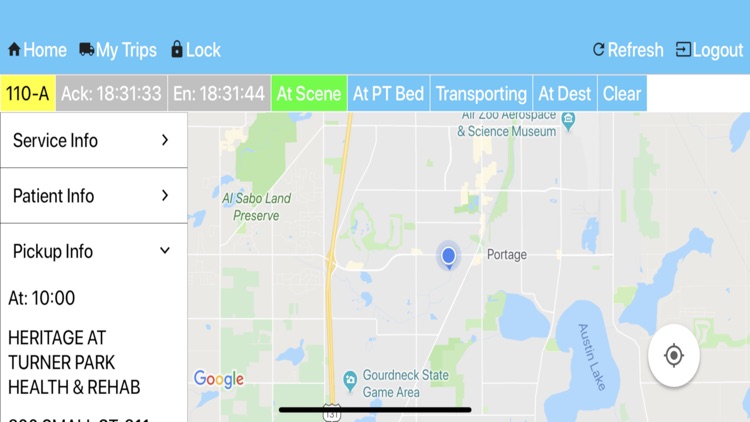This image displays a detailed navigation screenshot featuring multiple interface elements and map details. 

At the top left corner, three menu options are visible, each accompanied by a respective icon:
- "Home" with a house icon.
- "MyTrips" with a truck icon.
- "Lock" with a padlock icon.

On the extreme right of these options, there are two additional icons for refreshing the page and logging out.

Below these menu options, there are several tabs arranged horizontally. The first tab, highlighted with a yellow rectangle, reads "110-A." Next to it, there is a label "ACK: 18:31:33." The third column features a gray rectangle with the label "EN: 18:31:44." Moving further right, there is a bright neon green rectangle with the text "At Scene." Following this, there are several blue rectangles with different labels: "At PT Bed," "Transporting," "At Dest" (presumably "At Destination"), and "Clear."

Beneath these tabs, a map is displayed showcasing various locations, including:
- Al Sabo Land Preserve
- All 200 Airspace and Science
- Portage
- Girdock State Game Area
- Austin Lane

In the lower left-hand corner of the map, there is a small insignia and logo of Google.